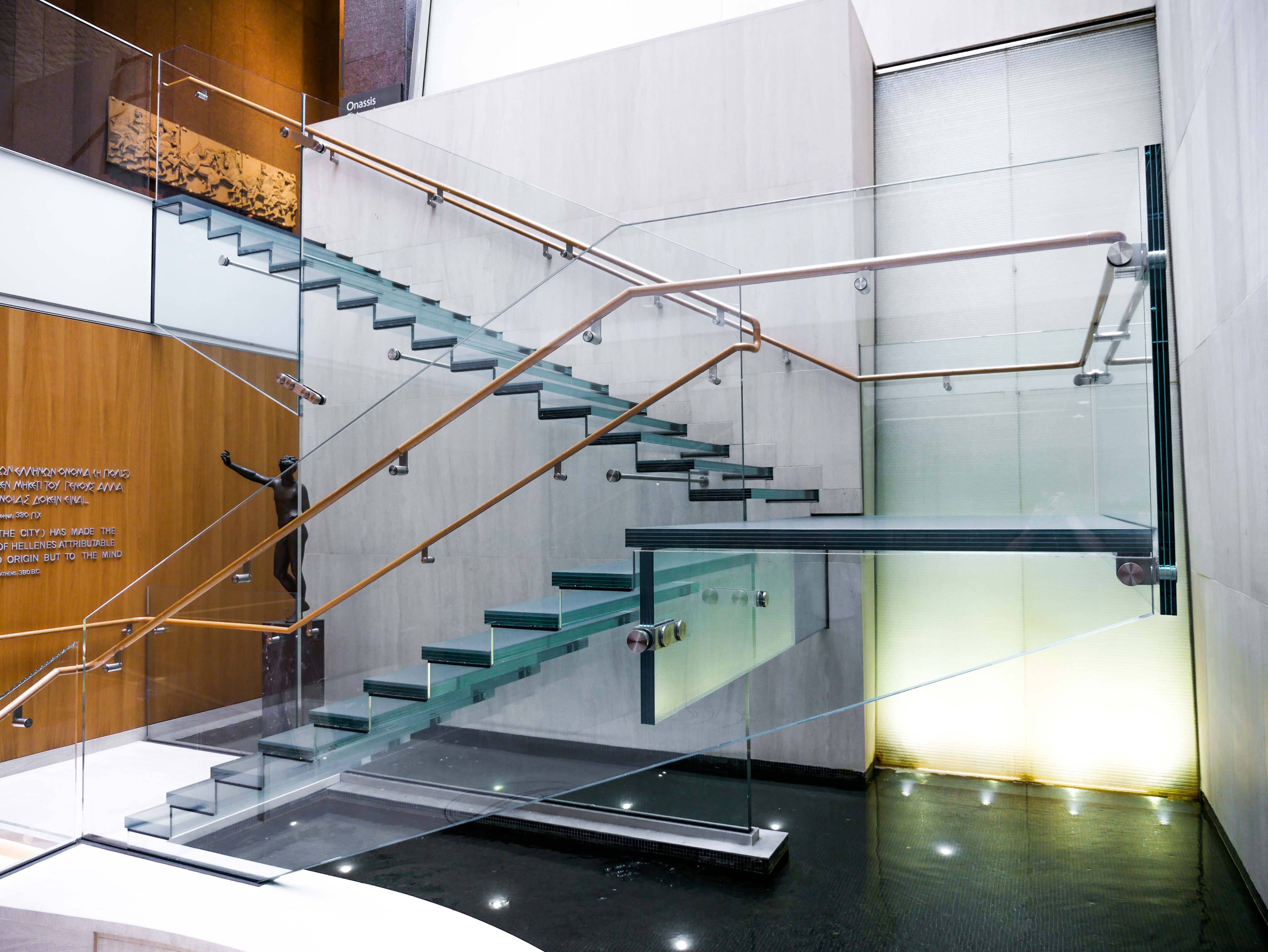The image depicts a modern staircase in an office building, characterized by its sophisticated design and materials. The staircase comprises two flights separated by a landing. The steps are crafted from clear glass, exhibiting a slight blue or green tint due to light reflection. The side railings are made of a transparent material such as lucite or acrylic and feature gold metal handrails. Underneath, the flooring is polished black marble illuminated by white or white-yellow lights.

Upon entering on the ground level, there's a wall with a wood grain finish that bears small, white-lettered writing, which is difficult to decipher. Adjacent to this wall, on the left, there is a statue of a man reaching out, positioned on a pedestal. Additionally, a wall on the right side of the staircase appears to be made of gray stone or slate, adding to the modern aesthetic of the space. Beneath the stairs, the detailed and well-lit environment contributes to the refined and professional atmosphere of the office building.